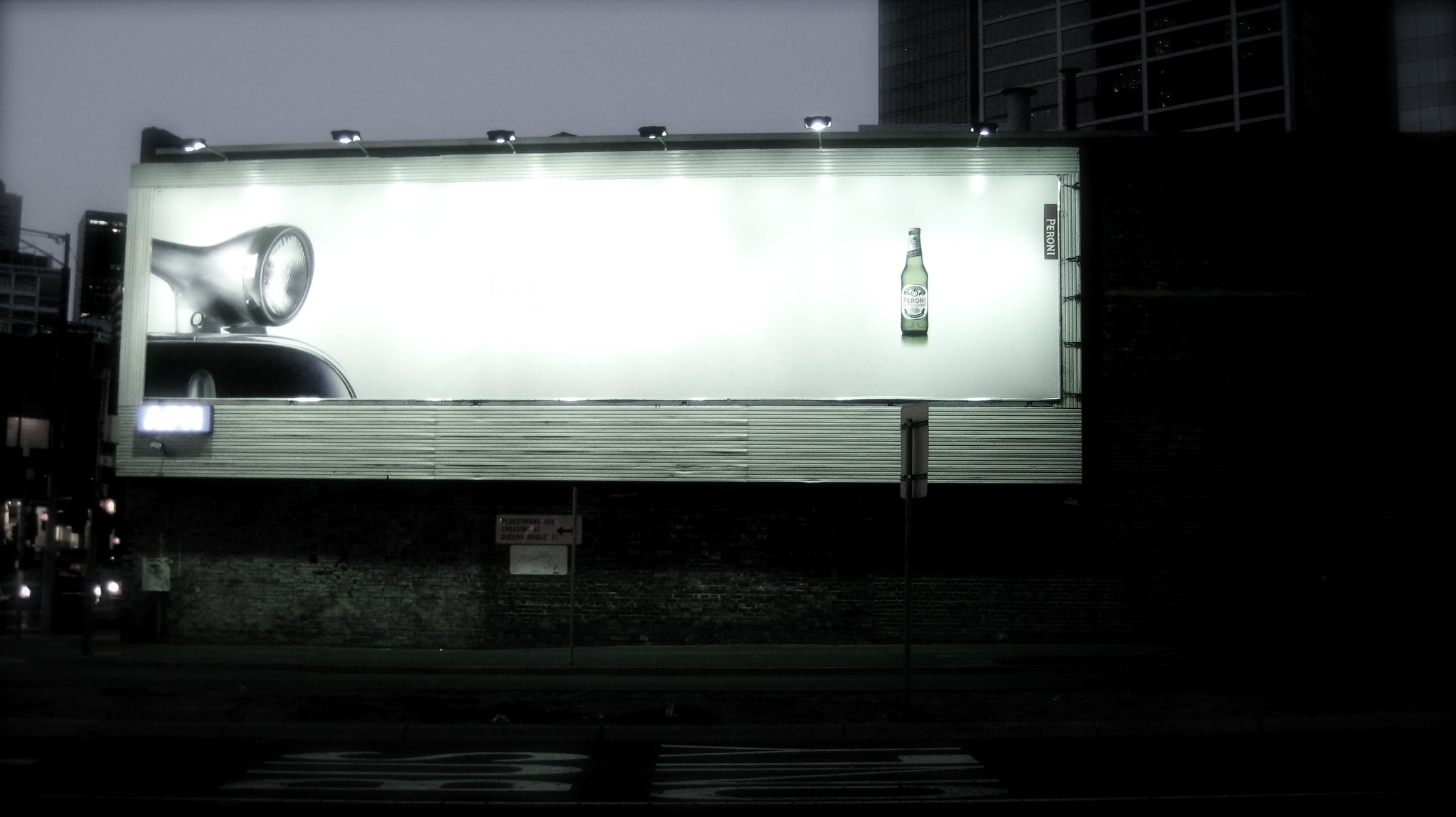In this nighttime color photograph, a high-rise building with dark glass windows and indistinguishable brick ends looms against a nearly gray sky. Dominating the scene is a large, rectangular billboard illuminated by six bright lights fixed on its top edge. The billboard displays a white-background image featuring a car with its headlights on, directing attention to a green bottle on the right side, possibly an alcoholic beverage. Below, a dark, nearly indistinguishable street stretches across the bottom of the picture, and the corners of the image are shrouded in darkness. To the left of the billboard, there's a partially visible object that looks like the top of a truck or SUV with a headlight on, though the details are murky due to poor lighting. The scene includes a small natural stone wall and what might be interpreted as a roof of a car or some other structure beneath.